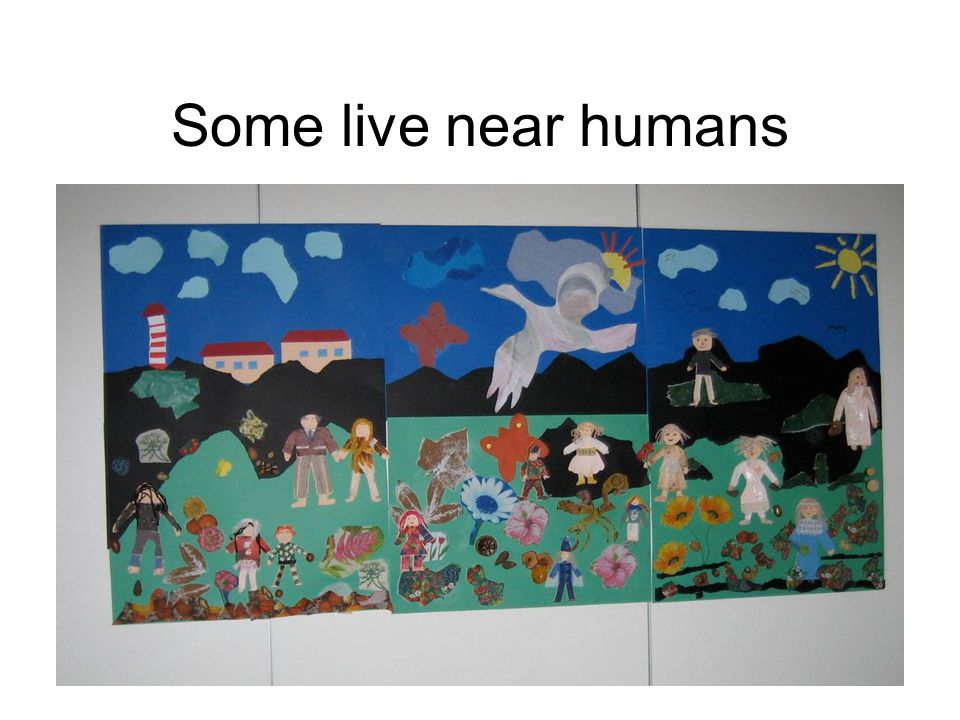The image titled "Some Live Near Humans" is a detailed, vibrant, and somewhat cartoony painting spread across three panels set against a white background. The painting features colorful outdoor scenes with a blue sky, white clouds, and two yellow suns—one in the middle panel and one in the top right corner. There is a white, ghost-like figure hovering in the sky. Below, a variety of people, including children, men, and women dressed in different clothes—mainly white dresses and brown suits—are depicted standing on a grassy field surrounded by flowers. In the background, there are black mountain silhouettes and buildings. The words "Some Live Near Humans" are in black Arial font at the top of the image. The panels, resembling pages taped together, create a cohesive, lively scene that seems reminiscent of a child's imaginative artwork.